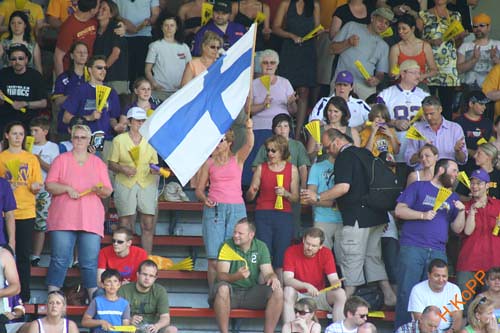This image captures a lively scene in the stands during what appears to be a sports competition, likely a soccer match. The crowd is seated on red bleachers against a white backdrop. The spectators are an eclectic mix, wearing various colored shirts, including purple, green, red, white, blue, pink, gray, and black. A prominent feature is the multitude of yellow fans with black writing, seemingly a giveaway from the event. The center of attention is a woman in a pink tank top, standing and proudly waving a white flag adorned with a blue cross, reminiscent of Finland's national flag. The atmosphere is vibrant, with fans energetically clapping, cheering, and moving their yellow fans. Additionally, a visible text, "H-COPP," suggests possible team or event branding. Overall, the image exudes the excitement and energy typical of a large, enthusiastic crowd at a major sports event.